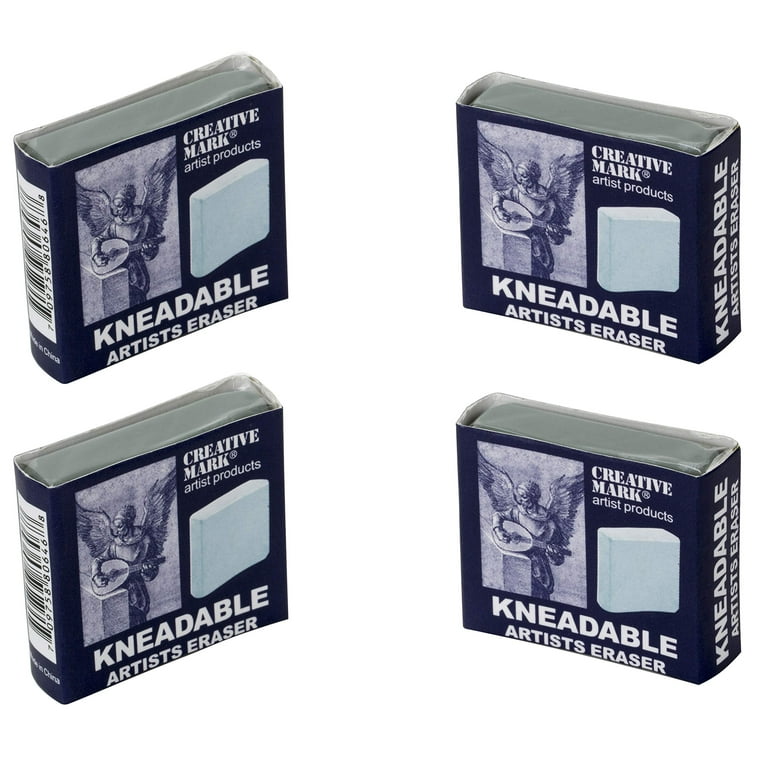This image showcases four kneadable artist erasers, each encased in a blue wrapper labeled "Kneadable Artist's Eraser" and "Creative Mark Artist Products." The wrappers feature an artistic depiction of an angel with wings, playing a stringed instrument that resembles a mandolin or guitar, drawn in blue pencil. Each eraser is a gray rectangular block and appears within its individual packaging, which includes a scanning barcode on the side. The erasers are arranged with two on the left and two on the right, all angled slightly towards the center, against a plain white background.